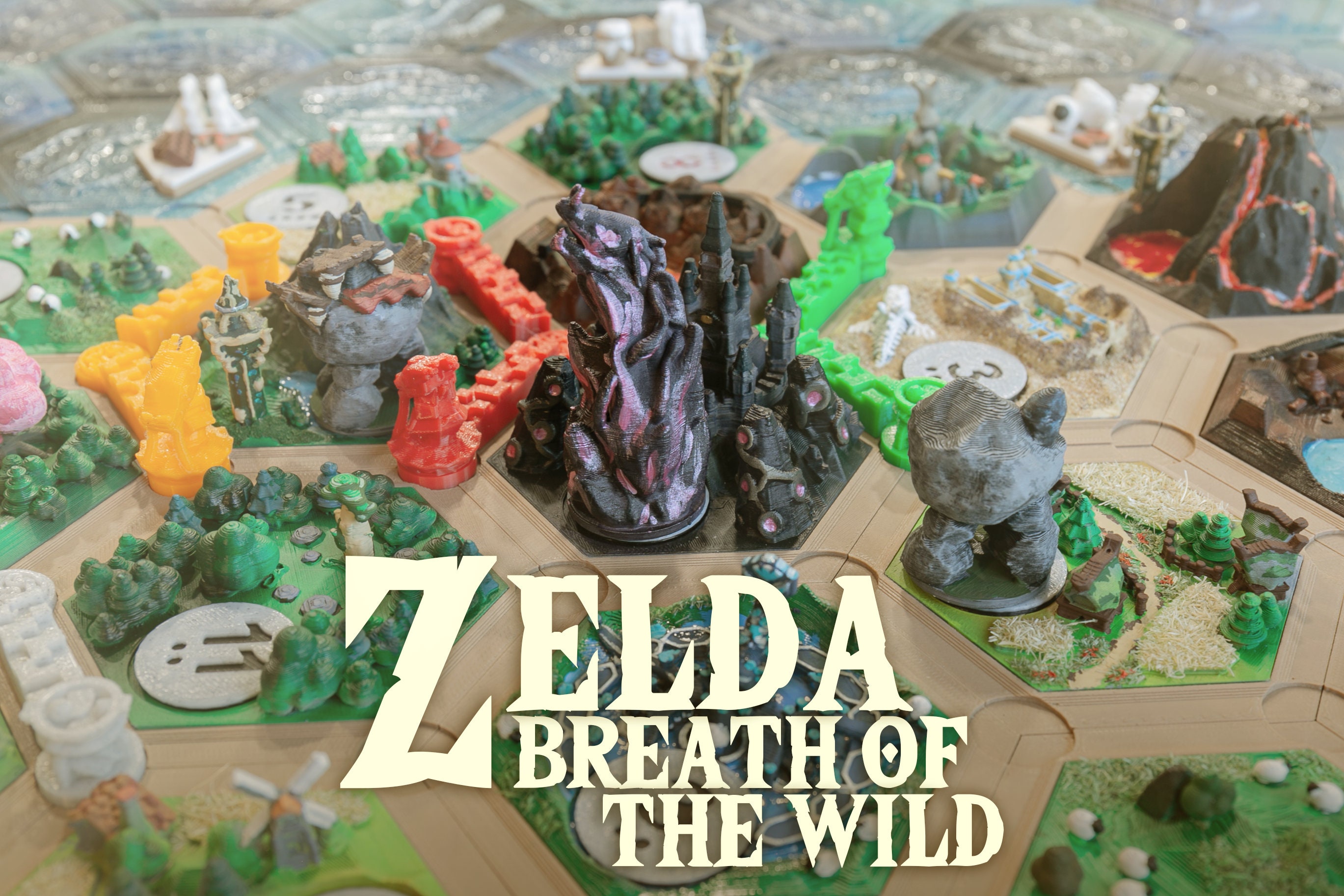This detailed image showcases a meticulously crafted 3D model or board game inspired by "Zelda: Breath of the Wild." Prominently displayed at the bottom in light yellow, official "Zelda" font text reads "Zelda: Breath of the Wild." The board is reminiscent of the classic game "Catan" but designed with distinctive elements from the Zelda universe. The landscape is composed of LEGO-like pieces, featuring a diverse terrain with rocky cliffs, grassy areas, pathways, and clusters of trees.

Positioned around the board are various numbered circular pieces, notably marked with numbers such as 11, 3, 5, and 8, placed strategically at certain distances from one another. The central area is dominated by a menacing, black castle surrounded by purple flames, likely representing a villainous fortress or base, possibly Hyrule Castle with Shadow Ganon or a similar antagonist. To the right, there's a towering mountain that may symbolize Death Mountain, alongside a rock creature on the center right, further enhancing the Hyrule landscape aesthetic.

Scattered across the board, there are various red and yellow towers and pieces that seem to form part of a defensive wall or boundary. The upper part of the model features water tiles, adding to the diversity of the terrain. This elaborate setup captures the essence of "Zelda: Breath of the Wild," transformed into a custom, Zelda-themed board game environment.